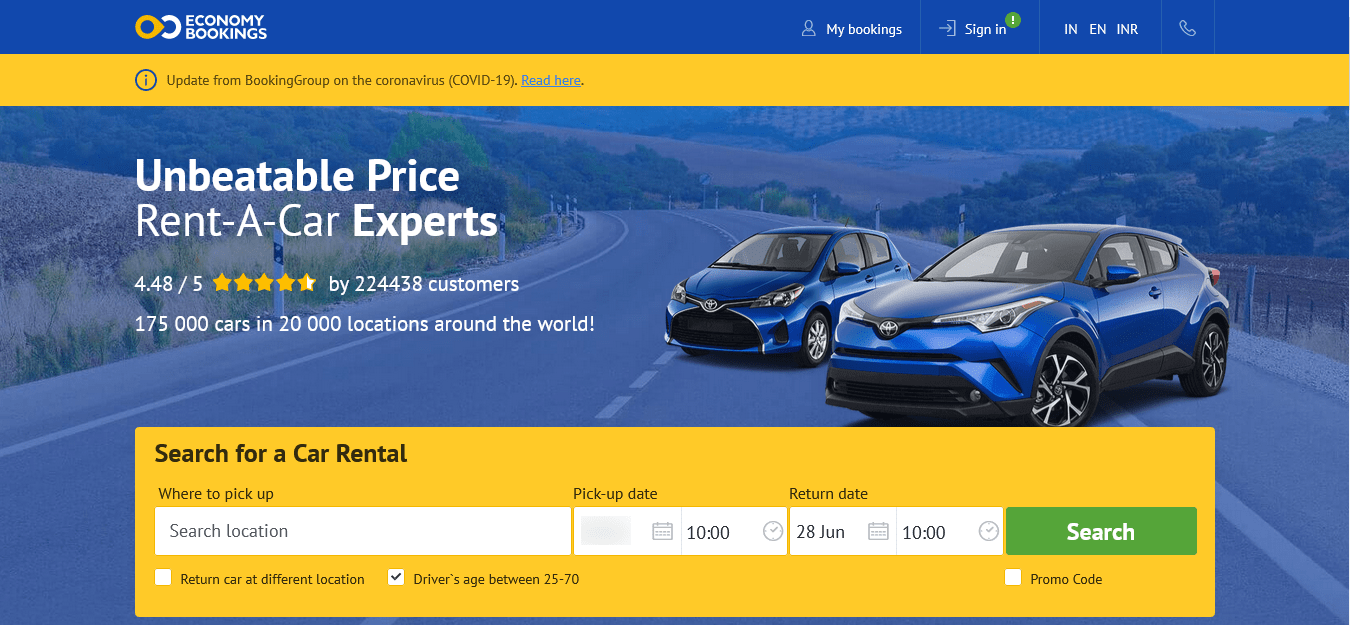This is a screenshot of the Economy Bookings website. 

At the top, there is a prominent bright dark blue banner. On the left side of the banner, the Economy Bookings logo is displayed. The logo features a gold-colored waypoint icon, which is circular on the left and tapers to a point on the right, with a white half-circle extending from it. Next to the logo, the words "Economy" (in all caps) and "Bookings" (in smaller caps) are stacked vertically, matching the logo's height. 

On the right side of the banner, several menu options are present. A pale blue icon resembling a person is followed by the text "My Bookings" in white. Next to this, a pale blue line break precedes an icon of an arrow pointing right, partially encased in a square missing its left side, with the words "Sign In" in white. Above this icon is a green circular icon with a white exclamation point. Another light bluish-gray line follows, creating a button that includes the language codes "IN" and "EN" and the currency code "INR" in white. Another light bluish-gray line follows, and a telephone icon is included, separated by additional bluish-gray lines.

Below this section, a gold banner with a blue circular icon containing an 'i' notes an important update: "Update from Booking Group on the Coronavirus (COVID-19)." Next to this update, a blue underlined "Read here" link is provided.

Further down, a large horizontal image of a road winding through hills and trees is visible. The road curves left, with metal poles and dashed lines indicating a highway. Two blue cars are angled towards the camera on the right.

On the left side of this image, large bold white letters state "UNBEATABLE PRICE." Below this, in smaller text, are the words "Rent-a-Car Experts," followed by a rating "4.48 / 5" from graphical gold stars and white fill. This rating is based on reviews from 224,438 customers. Below this, it mentions “175,000 cars in 20,000 locations around the world.”

At the bottom of the page, a gold box features the text “Search a Car Rental” in black. Below this, various search fields are laid out: "Where to pick up" with a gray text box for input, "Pick up date" with calendar and clock icons for selecting date and time, "Return date" with similar icons. June 28th and 10:00 AM are preselected. 

A green button labeled "Search" is at the bottom right, with a checkbox labeled “Return car to different location” below the search location input. Another checkbox, pre-selected, indicates "Driver's age between 25 to 70." Beneath the search button, there's an additional unchecked checkbox for a promo code.